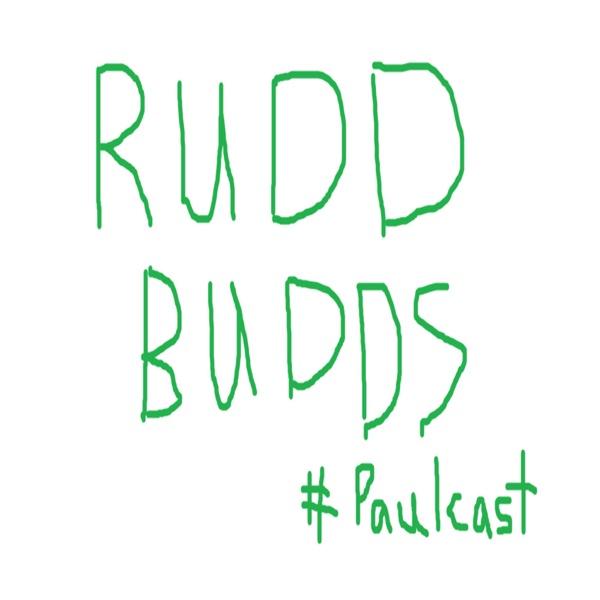This image features rough, hand-drawn lettering, likely created with paint or a similar application. The text is in large, dark green, uppercase letters against a solid white background. At the top, it reads "RUDD," followed by "BUDDS" in the middle. Positioned at the bottom right corner is the hashtag "#PaulCast." The handwriting is shaky and uneven, suggesting a homemade and low-quality aesthetic. There are no other objects or elements in the image, which gives it a stark, simplistic presentation.